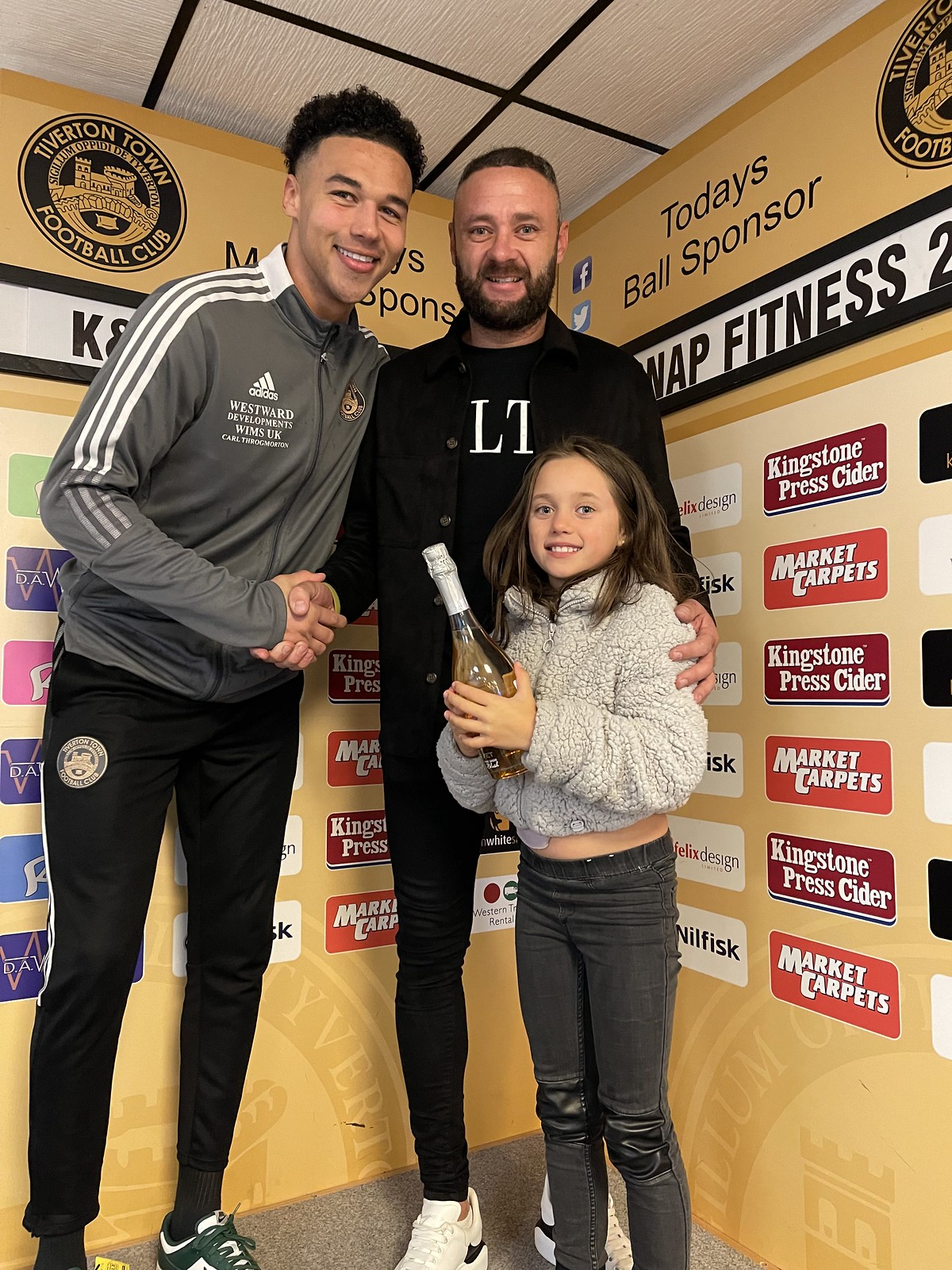The image depicts a lively scene in a room where two men are shaking hands while facing the camera, both smiling warmly. They appear to be in a corner of the room, with various texts and brand names painted on the walls behind them, organized into little square sections. Overhead, the ceiling seems rather low, causing the man on the left to lean somewhat to avoid hitting his head.

On the left stands a professional soccer player from Tiverton Town Football Club, identifiable by the club's emblem featuring a castle with a drawbridge, positioned at the top of the photo. This man is wearing casual sports attire, while the individual on the right, presumably a father, is dressed in a black unbuttoned shirt over a black t-shirt emblazoned with the letters "LT" in white. Directly in front of the father is a small child, his daughter, clad in a gray fake fur coat and gray jeans, holding what appears to be a bottle of champagne.